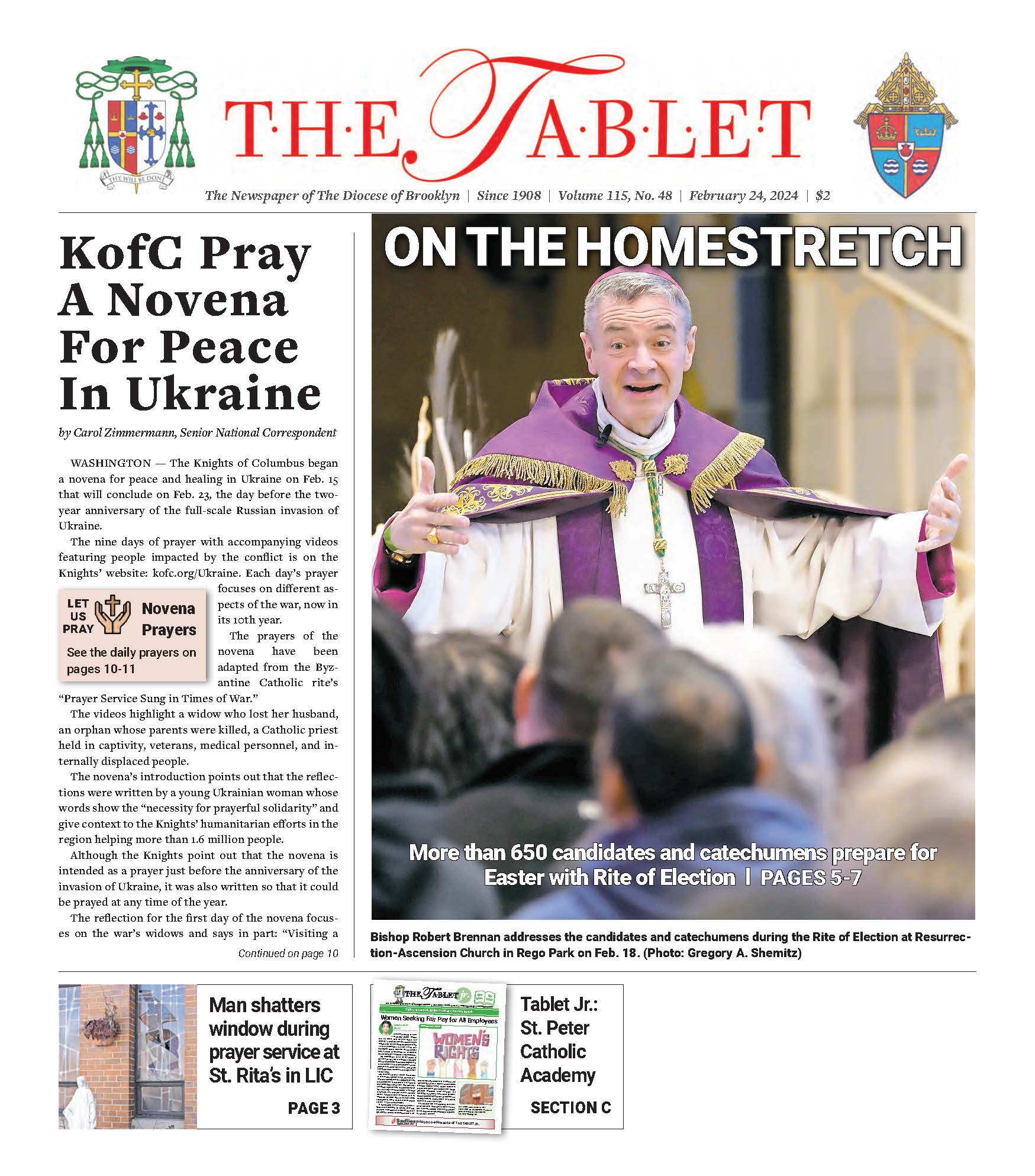The image depicts a newspaper page from "The Tablet," primarily featuring a white background. The newspaper's title, "THE TABLET," is prominently displayed in red capital letters at the top center, with an ornate script "T" in the word "Tablet." Flanking the title are two colorful crests, a distinct heraldic crest on the right and another emblematic crest on the left. Beneath the title, in smaller black text, it reads, "The Newspaper of the Diocese of Brooklyn Since 1908, Volume 115, Number 48, February 24th, 2024, $2."

Below the header, the page is divided into sections. On the left, there's a tall, narrow rectangle with an article titled, "KFC Pray a Novena for Peace in Ukraine," in bold black letters, authored by Carol Zimmerman, Senior National Correspondent. Within this article, a small light orange box with an illustration of praying hands invites readers to "Let us pray novena prayers," directing them to see the detailed prayers on pages 10 through 11.

Adjacent to the left pane, occupying about two-thirds of the remaining space, is a large photograph of a religious figure, identified as Bishop Robert Brennan. He is adorned in a white robe with purple cape and vestments, a cross around his neck, and a red cap on his head. His grayish hair is closely cropped, his mouth is open as if speaking, and his arms are outstretched. He faces the viewer directly, with blurred figures in the foreground listening to him. The caption in white type across the bottom of the photograph reads, "More than 650 candidates and catechumens prepare for Easter with the rite of election, pages 5 through 7." Below the image, in black type, it states, "Bishop Robert Brennan addresses the candidates and catechumens during the rite of election at Resurrection Ascension Church in Rego Park on February 18, photo by Gregory A. Schemetz." At the top of the photograph, within the image, in white block letters, the phrase "ON THE HOMESTRETCH" is displayed.

Further below, two smaller rectangles provide additional snippets; on the left is a notice stating, "Man shatters window during prayer service at St. Rita's and Lick, page 3," accompanied by a photograph of a broken window. On the right, another rectangle advertises "Tablet Junior, St. Peter Catholic Academy, section 3," with a small image of a mock-up newspaper beside the text.